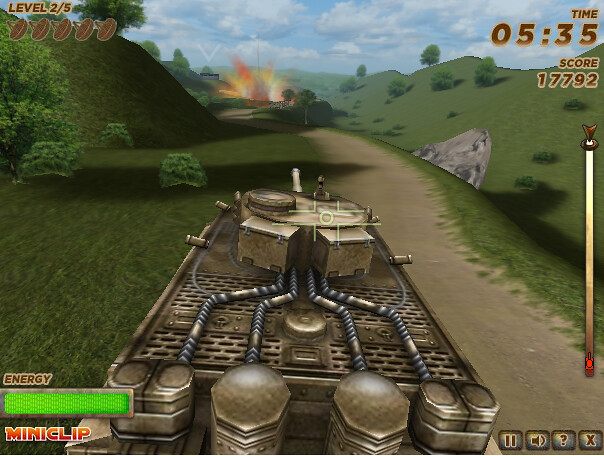The screenshot is from a game hosted on the Miniclip website. It features a tank, controlled by the player, situated on a dirt road surrounded by trees, bushes, rocks, and pixelated grass. Centered in the screen is a targeting reticle. In the distance, there is an explosion with visible flames, likely resulting from a recent shot fired by the tank. The top left corner displays "Level 2/5" with five satellite dish symbols. The upper right corner shows a timer set at 05:35 and a score of 17,792. A level progress bar on the right side highlights the tank's position near a gold marker, indicating its progress. The lower left corner contains a full energy bar glowing bright green, the word "Energy," and the Miniclip logo in red. The bottom right corner offers game controls: a pause button, a volume button, a question mark button for help, and an X button to presumably exit the game. The graphics reflect a typical Miniclip game's low resolution, adding a nostalgic charm to the scene.